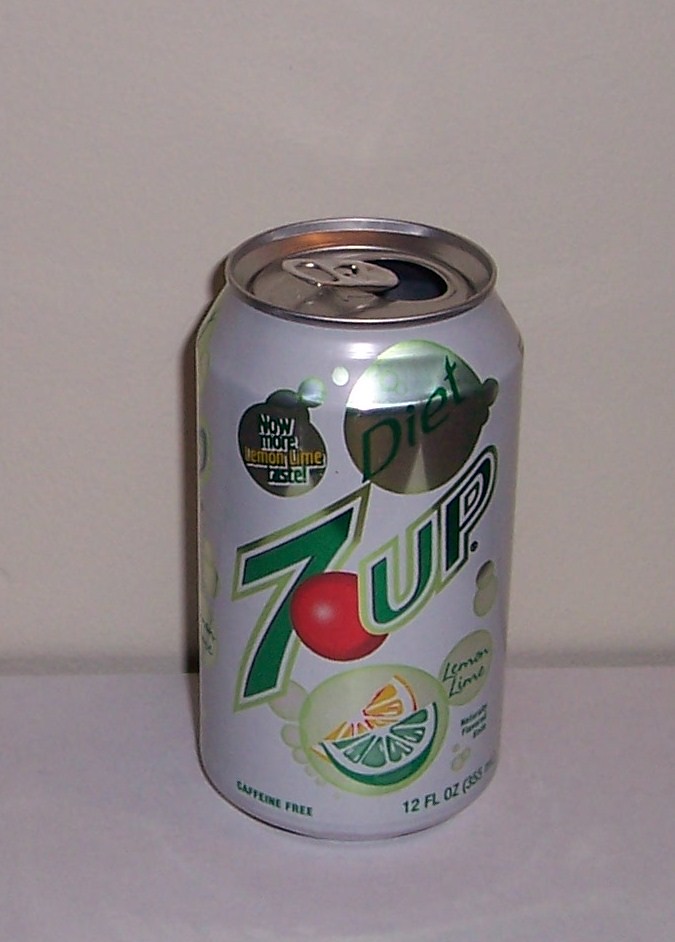The image features a countertop with a grayish-beige hue, set against a coordinated beige background. Resting on this counter is an aluminum can of soda, prominently displayed at the center of the frame. The can has already been opened, with the pop ring still attached. Its color is a very light gray, almost silver, creating a contrast with the bold green lettering that adorns it. In the center of the can's front, the number "7" and the letters "UP" are written in large, vivid green font. Above this central text, there is a circular emblem also in green, inside which the word "DIET" is clearly visible, though the remaining letters within this emblem are too obscured or small to be legible. The lighting in the image highlights the reflective quality of the aluminum, giving the can a fresh, slightly glossy appearance.